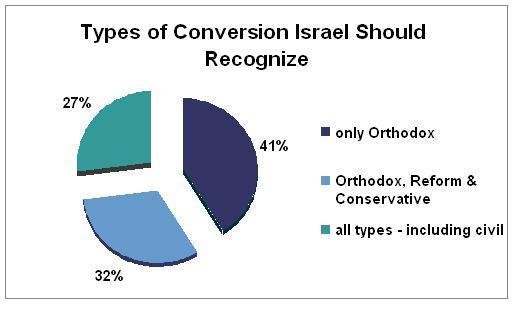The image features a detailed, computer-generated pie chart titled "Types of Conversion Israel Should Recognize" in black text at the top center. The pie chart, approximately 4 inches tall and 6 inches wide, is set against a white background with a black border. It consists of three color-coded slices, each indicating different perspectives on types of conversion. The largest slice, comprising 41% in dark purple, represents the viewpoint that only Orthodox conversions should be recognized. The second slice, 32% in light blue, encompasses Orthodox, Reform, and Conservative conversions. The final slice, 27% in teal, includes all types of conversions, including civil. On the right side of the chart, these color codes and corresponding percentages are clearly explained, underlining the varying opinions on the matter.